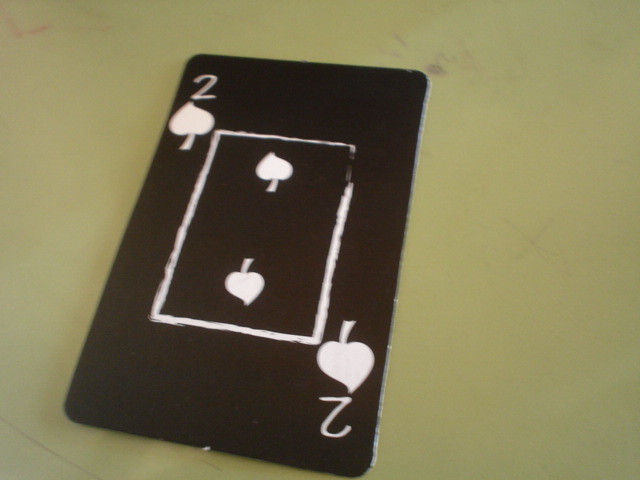A slightly diagonal, black two of spades playing card occupies the center of a brownish-beige background in this photograph. The card, featuring prominent white text and numbers, tilts towards the picture's right side. Its bottom edge touches the lower center of the frame, while the top edge angles gently upwards and rightward. Surrounding the card, the table surface bears a few greyish smudges, adding texture to the scene. Although the card is somewhat blurry, the design details are discernible. A notable feature of the card is its handmade appearance, emphasized by a white rectangular border that is intentionally broken at the edges, suggesting a unique, custom-crafted origin.